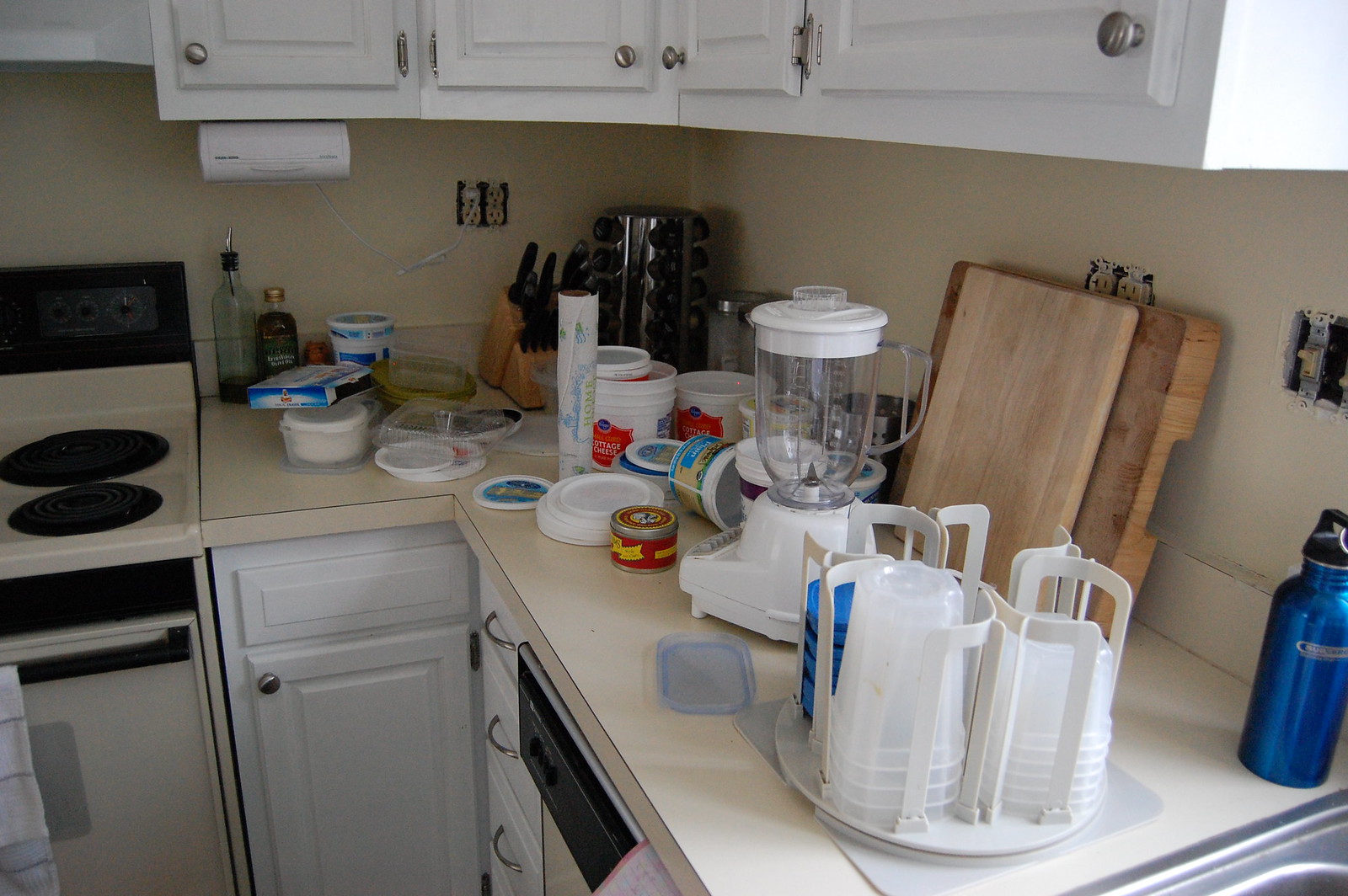A photograph captures the corner of a well-used kitchen. The countertops, fashioned from pale ivory Formica, are cluttered with an array of dishes, cutting boards, storage tubs, and a knife block. A sleek blender and various other kitchen essentials further populate the space. The cabinets, pristinely white with silver fixtures, complement the walls that share the same yellowish ivory hue as the countertops. Central to the scene is an older model electric stove featuring spiral heating elements. Adjacent to it, a metal sink gleams under the kitchen light, bordered by a dishwasher. In the corner, partially obscured by the surrounding items, lies an indistinct metal object. Notably, the outlets along the walls lack their covers, revealing a minor oversight in an otherwise functional kitchen space.